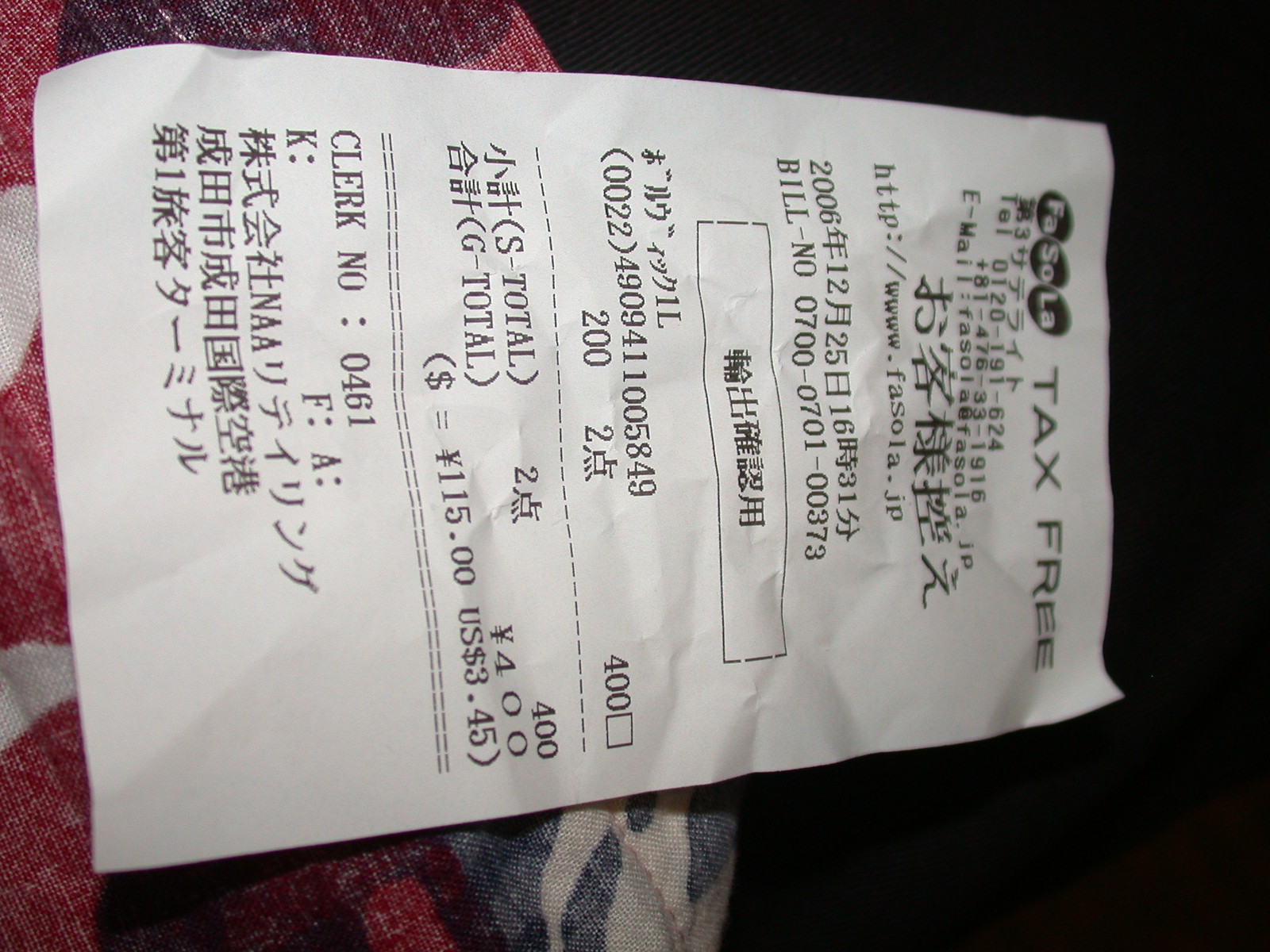This image features a receipt positioned sideways against a backdrop with distinct contrasting elements. The right side of the background is solid black, while the left side showcases a piece of fabric adorned with red, white, and blue colors, possibly resembling a flag. The receipt itself is white with black printed text. At the top, which is situated at the top right of the image due to its sideways orientation, the text "F-A-S-O-L-A, tax free" is prominently displayed. Directly below this, there are Japanese characters, followed by the string "TEL 0120-191-620". The receipt appears to be well-lit, making the text easily readable despite its sideways placement.